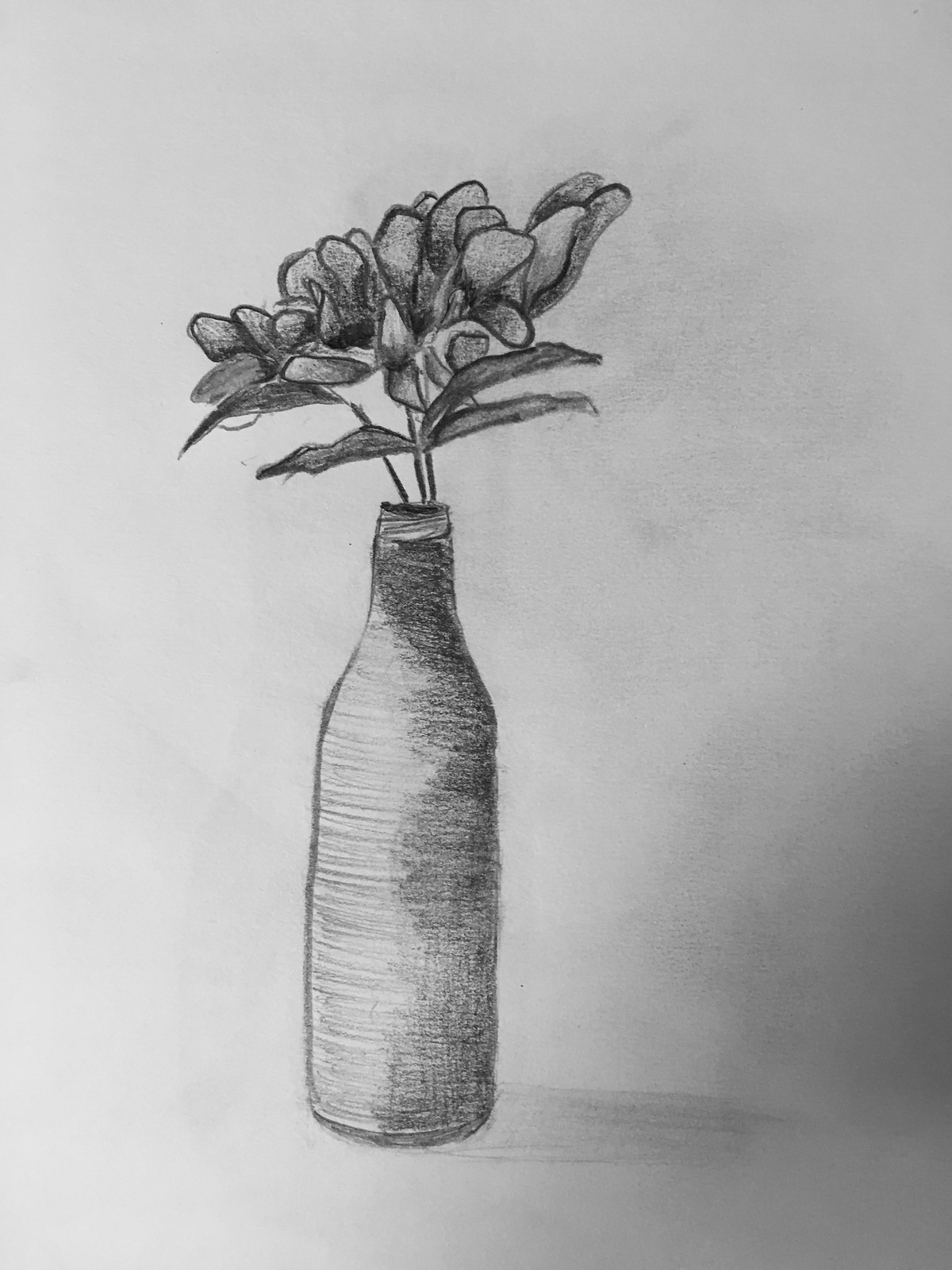This detailed pencil drawing on white art paper depicts a bottle-shaped vase. The vase is meticulously shaded, with the right side and the ground behind it featuring deliberate shadowing to create a sense of depth. Emerging from the neck of the vase are three detailed stems, each supporting flowers and four elongated leaves. The flowers are clustered at the top, portrayed in a uniformly dark pencil shade, contrasting with the more nuanced shading of the vase itself. One of the flowers in the background appears to have numerous petals and is on the verge of blooming, adding a dynamic element to the composition. The sketch thoughtfully combines light and shadow to emphasize the texture and form of both the vase and the organic elements sprouting from it.